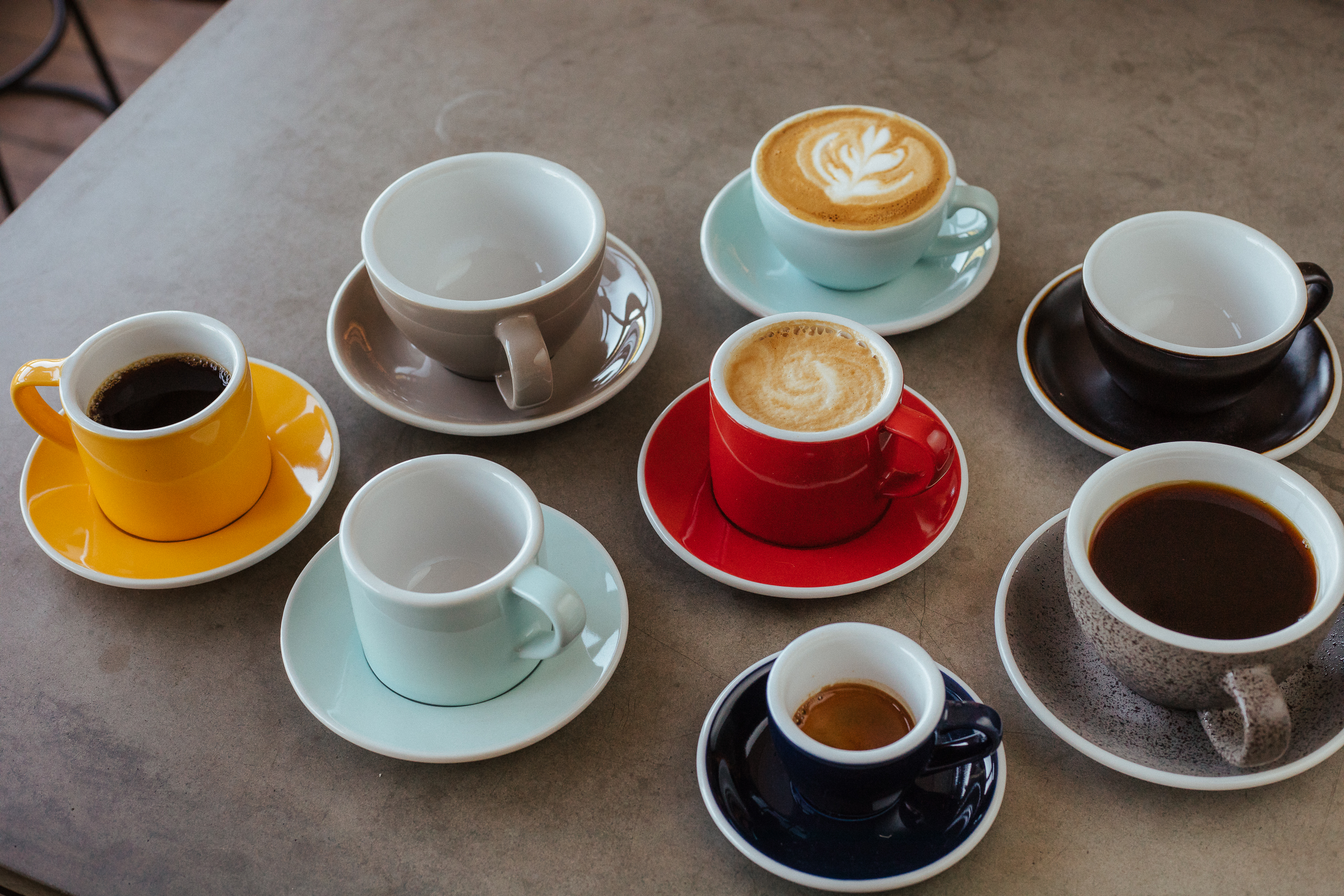In this overhead photograph, a section of a gray tabletop is visible along the top edge, with a glimpse of a wooden floor and possibly a metal chair in the upper left corner. Arranged on the table are eight pairs of cups and matching saucers, each in different colors: yellow, light blue, two shades of gray, white, red, black, and dotted brown. The cups and saucers are organized from the middle left of the image, arcing up slightly to the right, and then scattered across the frame. Some cups are empty, revealing their white interiors, while others contain beverages, predominantly coffee or tea, with two displaying intricate foam patterns resembling flowers. Specifically, the arrangement includes:
- A yellow cup on a yellow saucer with some coffee.
- A gray cup on a matching gray saucer, empty inside.
- A white cup on a white saucer, filled with coffee adorned with a white flower foam design.
- A black cup on a black saucer, empty inside, near the right edge of the image.
- A gray speckled cup on a matching saucer filled nearly to the brim with coffee.
- A red cup on a red saucer, partially filled, with a frothy coffee and a white design.
- A blue cup on a blue saucer containing coffee with a bit of cream.
- Another white cup on a white saucer, empty, positioned towards the bottom edge.

There are three cups that are empty and five filled, contributing a varied visual and textural composition to the scene.